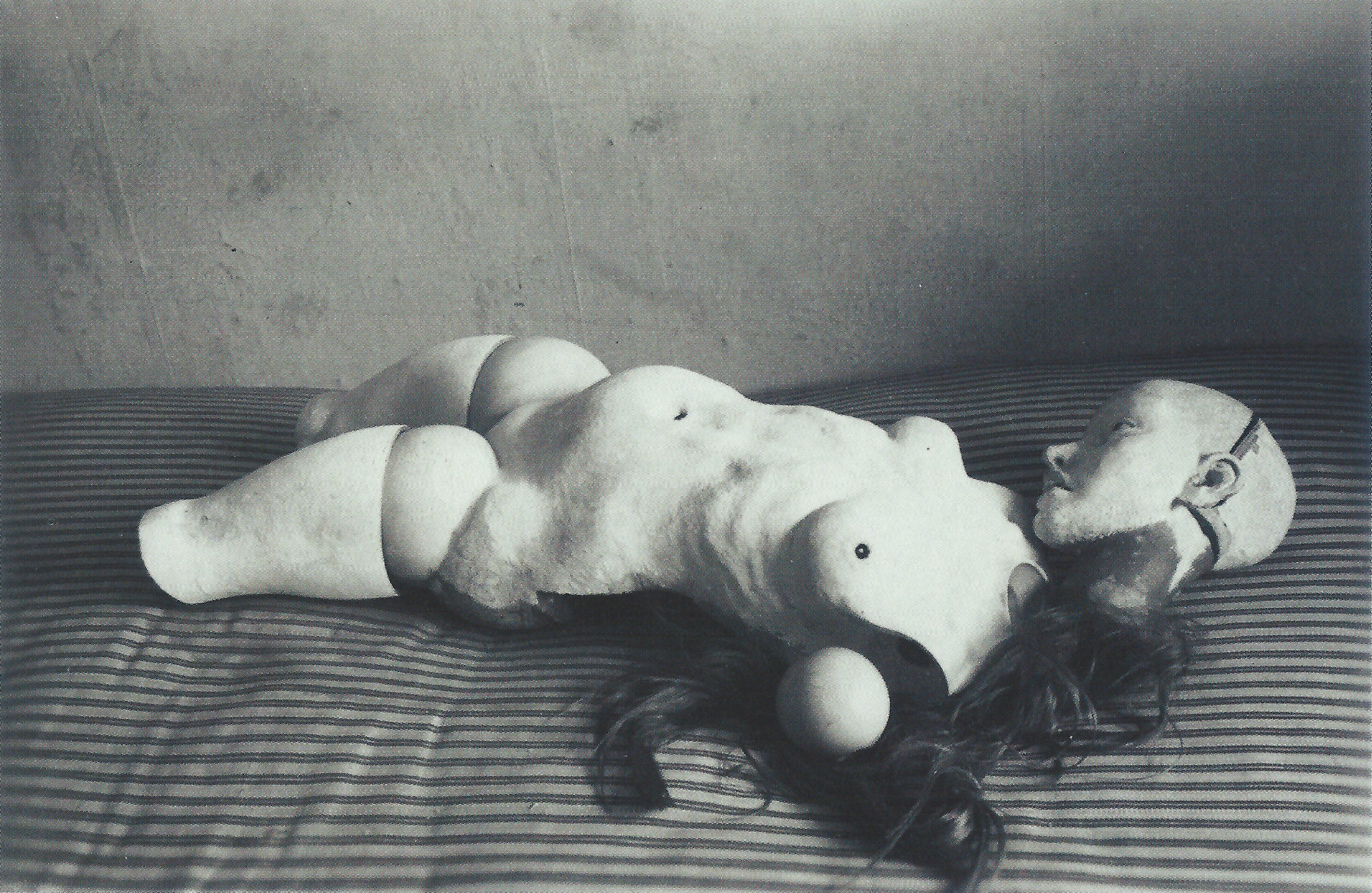This black-and-white photograph depicts a disturbing scene of a disassembled mannequin or sculpture of a naked female body. The body is laid out on a striped gray and dark gray mattress with a light gray, slightly worn and dirty wall in the background. The figure's head, which features a visible crack in the skull and remnants of chipped paint, is detached and positioned on the mattress facing the torso. The hair, a dark and long wig, is partially visible beneath where the neck would have been. The torso is accompanied by upper thighs and knees, but the legs are severed below the knees. The figure lacks arms, though a notable joint or ball is visible where one shoulder would have been. The overall composition highlights the unsettling fragmentation and decay of the mannequin, accentuated by the stark and barren setting. No text is present in the image.